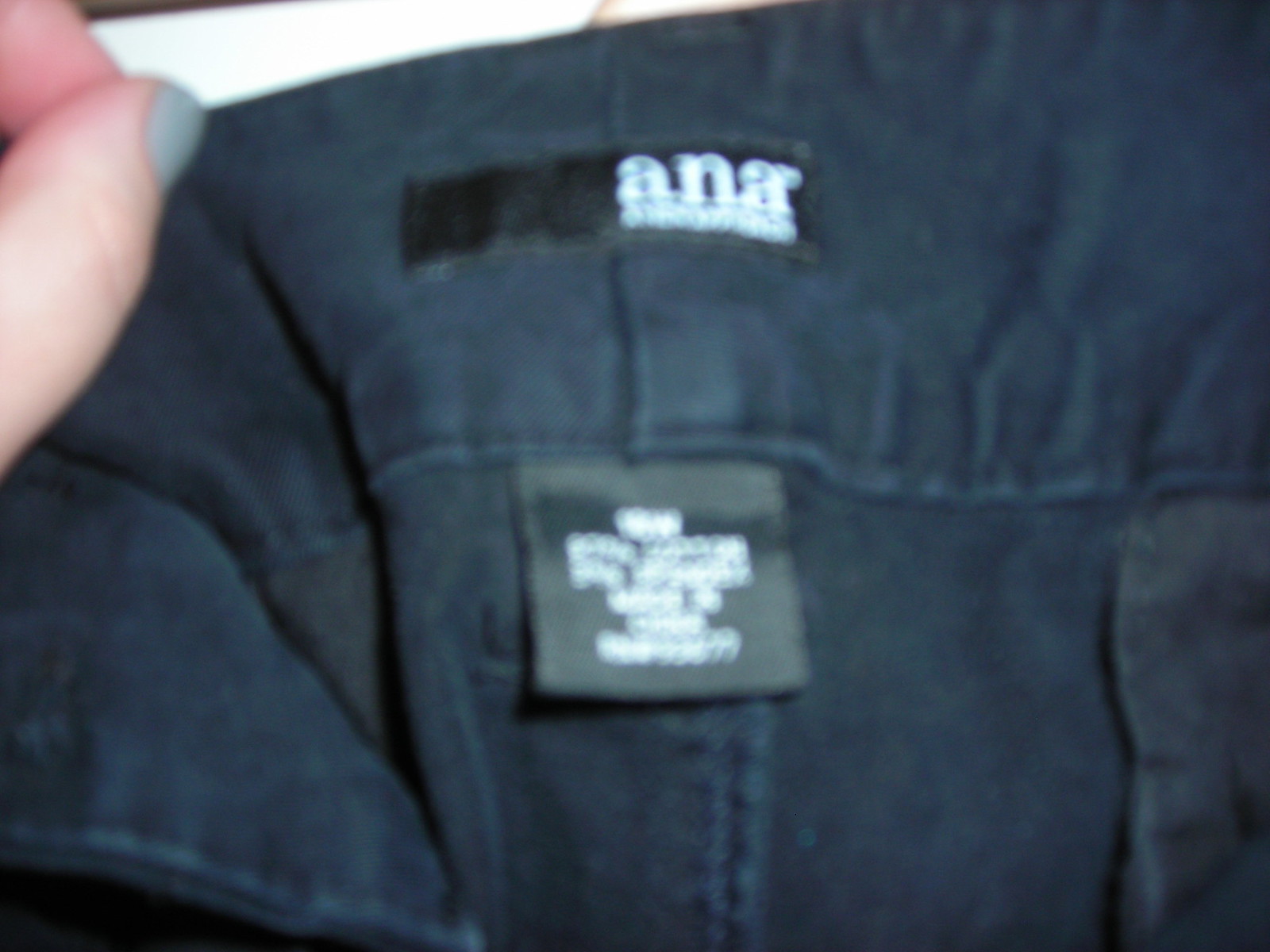This blurry photograph seems to capture a piece of dark blue clothing, possibly a shirt or jacket. In the upper right-hand corner, a person's thumb with a gray-painted fingernail is visible. At the top of the garment, a black rectangular tag with white letters "A-N-A" can be seen, though the text underneath is too blurred to decipher. Further down, a black tag appears, which seems to display a number and possibly the letter "W." The tag also contains text, including what seems to be the words "Made in China," though this part remains indistinct due to the blurriness.